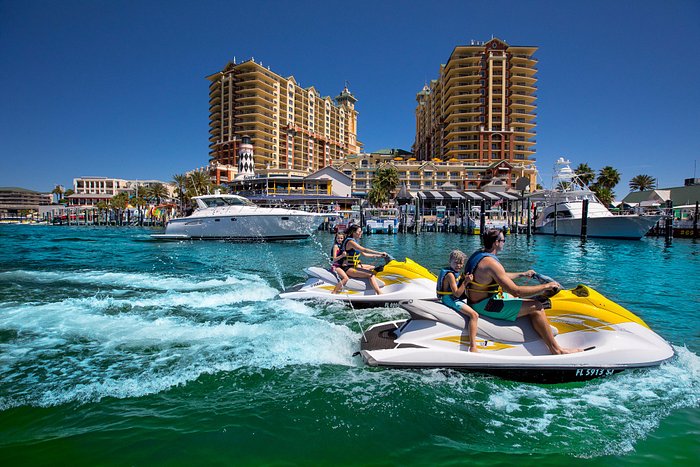This modern outdoor photograph captures a vibrant family adventure on the water, set against an urban backdrop. The foreground is dominated by two yellow and white jet skis, each occupied by family members. Closest to the camera, a man in aqua-colored swim trunks and a blue life jacket steers the first jet ski, with a young boy in matching aqua shorts and a blue life jacket seated behind him. Beside them, on a second jet ski, a woman in a black swimsuit and blue life jacket navigates with a young girl in a pink swimsuit and blue life jacket riding pillion. The water beneath them churns with movement, creating wakes that accentuate the sense of speed and excitement. In the background, a marina crowded with boats and yachts stretches out in front of towering condo buildings, beige and white with numerous windows, rising against a clear blue sky, lending a contemporary, urban feel to the scene.